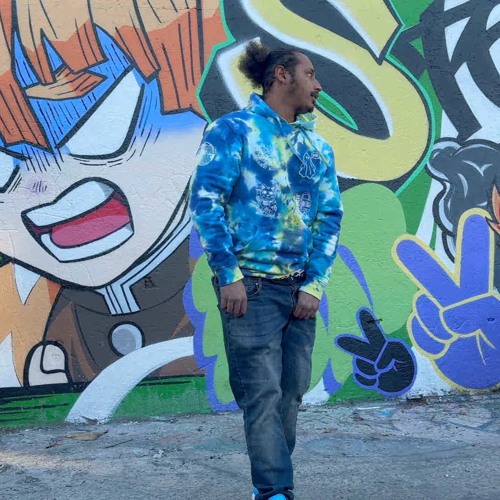A young Black man is captured standing on a sidewalk, gazing contemplatively to the right. He’s dressed in a blue tie-dye hoodie accented with splashes of yellow, white, and hints of green, paired with blue jeans. His hair is neatly pulled back into a ponytail. Behind him, a graffiti-covered wall bursts with colors and imagery, dominated by an anime character from Demon Slayer. The character features striking details: white eyes with a blue area above them, orange hair, a brown shirt, and a snarling expression with exposed teeth and visible tongue, indicating anger or confusion. The vibrant background also includes a large yellow letter 'S' on a green backdrop and several peace symbols—one blue with a yellow outline and another black with a blue outline. Although the scene's lighting is somewhat muted, giving a cloudy and subdued atmosphere, the combination of the man's attire and the vibrant street art creates a striking visual contrast.